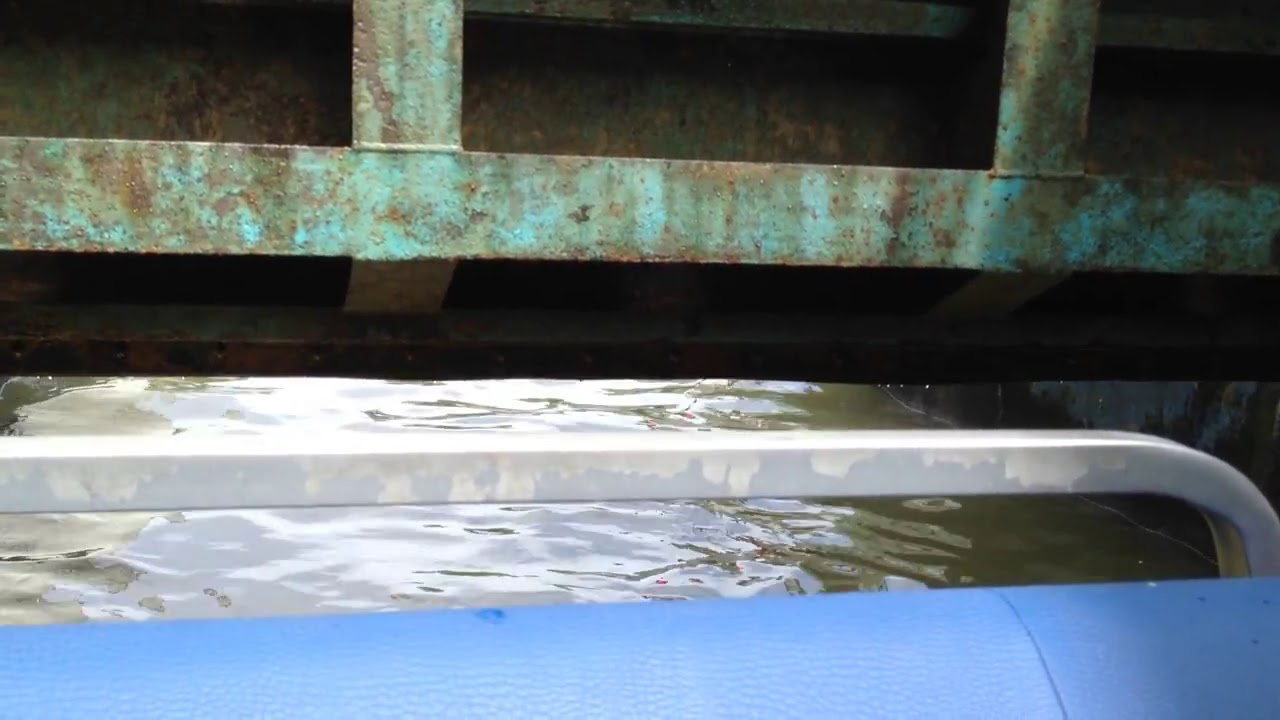The image depicts a scene from a boat traveling through a narrow, possibly industrial, waterway such as a canal or drainage spot. At the top of the rectangular frame, a rusty metal gate can be seen, initially painted green but now showing signs of wear and corrosion, with two supporting pillars and a mesh in between. Below this gate, the shadow highlights the murky, rippled water, further revealing reflections of a daytime sky with clouds. In the lower part of the image, a bright blue surface, likely the leathery seat of the boat, is visible, along with a metal bar that rises just a few inches above the seat. This bar looks weathered and wouldn't suffice as a safety barrier. The industrial structure, possibly an overhang or part of a bridge, dominates the upper background, showcasing a mix of turquoise and brownish rust due to prolonged exposure to the elements. The composition suggests the boat is either passing under or alongside this deteriorated overhang, capturing both the rugged industrial atmosphere and the boat's dilapidated elements.